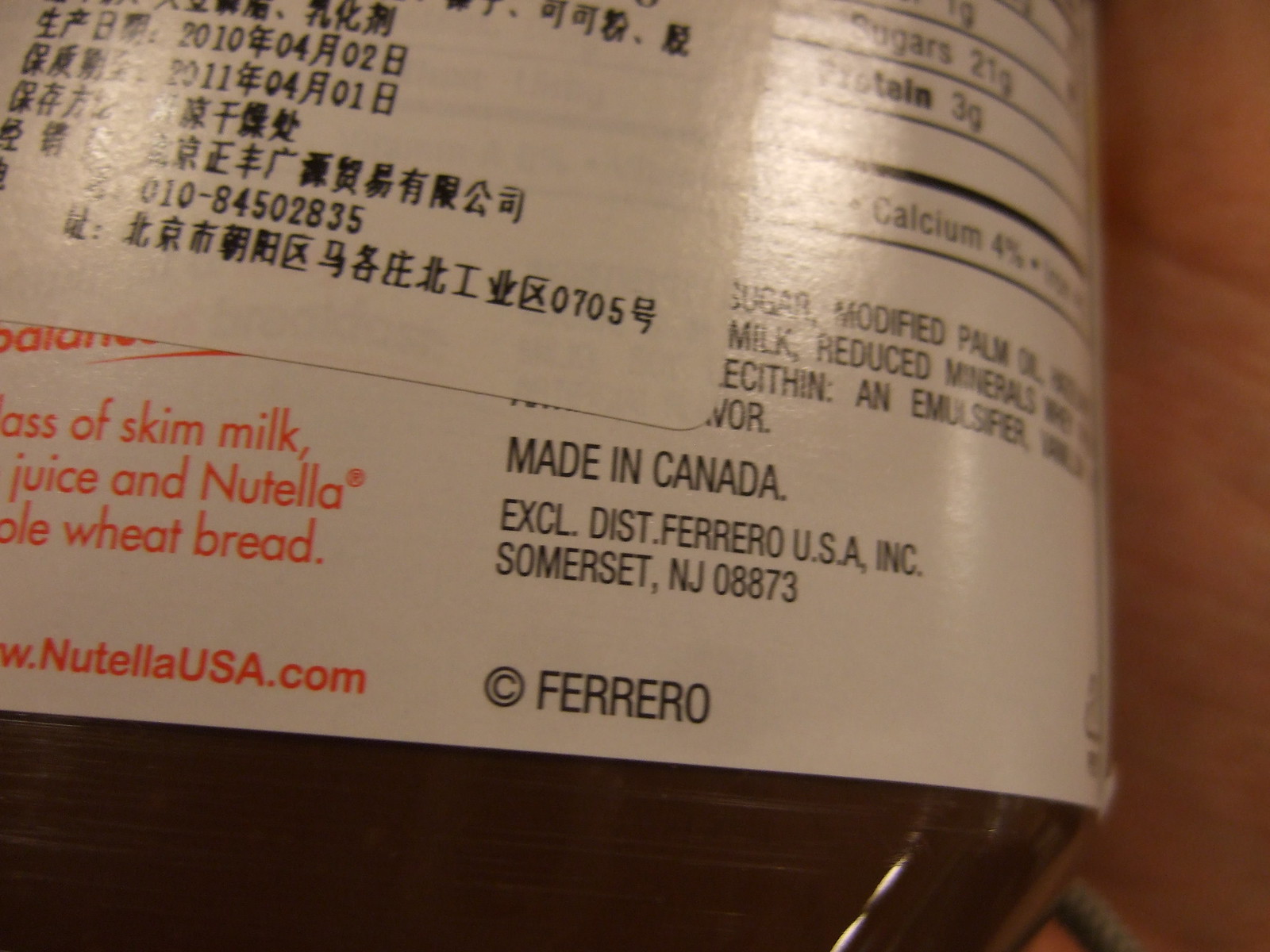This detailed image depicts the back of a Nutella jar, identified as a Ferrero product, with notable features. Although Nutella typically caters to an American audience with standard English labeling, this particular jar stands out due to an additional white label featuring Japanese characters and possibly Chinese characters, indicating it is likely an imported product. The original product label, stating "Made in Canada" and "Distributed by New Jersey," is visible beneath this extra label. The transparent sections of the container reveal the chocolate brown Nutella inside. The label displays parts of the ingredients and nutrition facts, mentioning elements like "skim milk," "whole wheat bread," and "modified palm oil." The text also highlights “NutellaUSA.com” as the official website. The jar rests on a wooden table, with the edge of the table barely visible on the right side, and no other items are present in the image.